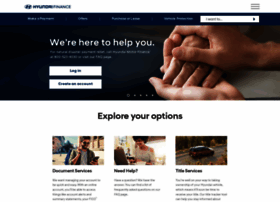This image showcases a website page displayed in portrait orientation on a white background, with no defined borders. At the top, there's a horizontal white bar featuring a circular logo with an H-shape inside, presented in green font on a white background, though the precise details are somewhat unclear. Next to the logo is a bolded word, indistinct due to blurriness, followed by a term that resembles "France." The top right corner houses a hamburger menu icon.

Below this, a dark blue horizontal bar spans the width of the page, containing a few options. The specific details of the text on the left are unclear, but there are two white clickable options positioned on the right of this bar. Adjacent to these options, aligned horizontally, is a white search bar.

Further down, against the white background, there is a section featuring a blue "Login" button at the top, with a "Create Account" button in a matching blue font below it. Beneath these buttons are three dots, followed by a header that reads "Explore Your Options." Directly under this header are three blurred images arranged from right to left, the specifics of which are unfortunately too indistinct to decipher.